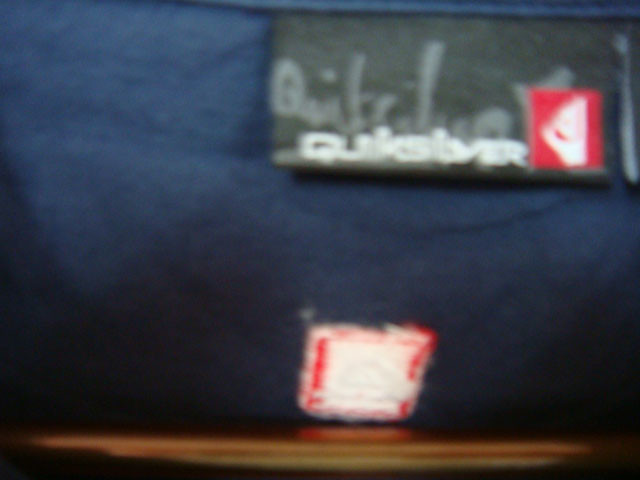This photograph, although blurred, captures a detailed scene with a blue-draped cloth serving as the background. At the bottom of the image, there is a wooden table with a brown finish. Positioned on the table is a circular red object. Resting on this object is a white square, partially rimmed in red. Above this setup, a dark gray banner with lighter gray writing is visible, possibly spelling "Q-U-I-T-E-L-L" or "A-U," though the text is partially cut off and hard to decipher. Additionally, a red page sits on a ledge, featuring a sideways triangle and further indistinguishable text, including "Q-U-T."